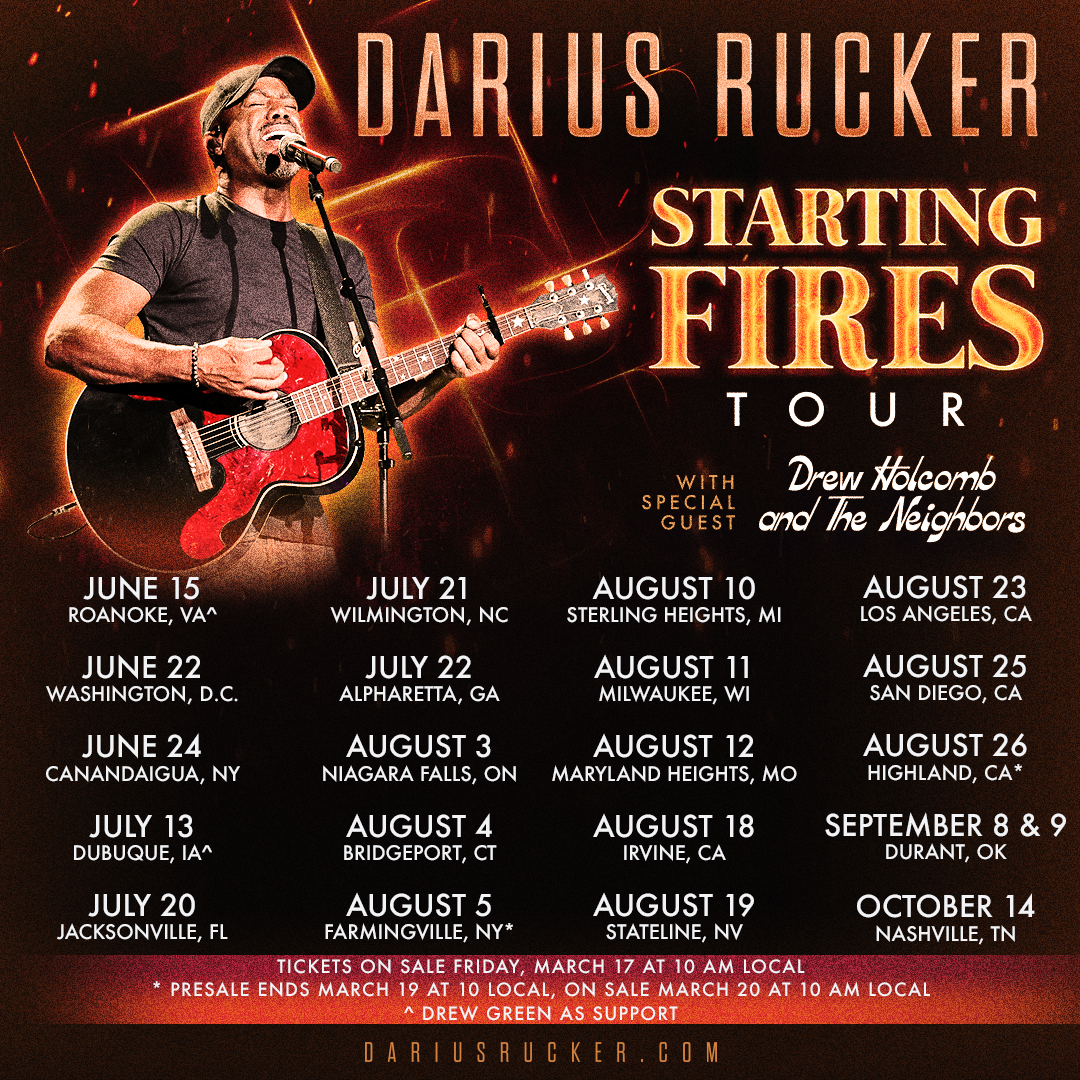This is a detailed flyer for Darius Rucker's "Starting Fires Tour." The flyer features a prominent image of Darius Rucker on the top left, passionately playing guitar and singing into a microphone, with his eyes closed. He is wearing a hat and a black t-shirt, immersed in his performance, set against a dark background with a red glowing effect.

The tour includes special guests Drew Holcomb and the Neighbors, and Drew Green for support on various dates. The extensive list of tour dates stretches from June 15th in Roanoke, VA, through October 14th in Nashville, TN, with performances in cities like Washington, D.C., New York, Dubuque, IA, Wilmington, NC, Niagara Falls, CT, MI, WI, MO, CA, NV, and more.

Tickets go on sale on Friday, March 17th at 10 a.m. local time, with a pre-sale ending on March 19th at 10 a.m. local time, and general sales reopening on March 20th at 10 a.m. local time. For more information, fans are directed to visit DariusRucker.com.